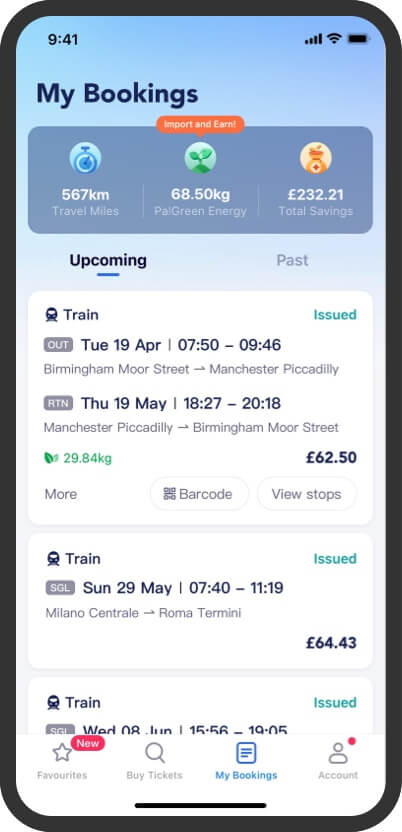**Caption:**

The image depicts a simulated cell phone screen that resembles a design you might see in an advertisement. The screen has a black border and a background gradient of blue and white. At the very top, the status bar displays the time "9:41" in black, alongside icons for Wi-Fi, battery level, and signal strength.

Below the status bar, the heading "My Bookings" is written in black. A prominent blue box occupies the center of the screen, containing several icons and statistics in white text. At the top of this blue box, an orange section displays the text "Import and Earn."

Within the blue box, there are three circular icons with their corresponding data:
1. A blue circle with a stopwatch icon indicating "567 kilometers traveled."
2. A green circle with a plant icon signifying "68.50 kilograms of green energy" saved.
3. A gold circle with a money bag icon denoting "232.21 pounds total savings."

Further down the screen, the interface is divided into two tabs titled "Upcoming" and "Past," with "Upcoming" highlighted by a blue underline.

Under the "Upcoming" section:
- A train icon accompanies the text for a journey scheduled on Tuesday, April 19th, from 7:50 to 9:46 AM, traveling from Birmingham Moor Street to Manchester Piccadilly. Additional details include a return trip on Thursday, May 19th, from 6:27 to 8:18 PM. The text shows travel metrics: "29.84 kilograms" in green, "62.50 pounds" in navy, a barcode icon, and "View Stops" in gray text.
- Another train journey is listed for Sunday, May 29th, from 7:40 to 11:19 AM, traveling from Milano Centrale to Roma Termini, marked with "Issued" in teal and the fare "64.43 pounds" in navy.
- A final journey scheduled for Wednesday, June 8th, from 3:56 to 7:05 PM, includes a "Issued" status in teal, and fare details "64.43 pounds" in navy.

At the bottom of the screen, several icons are displayed in gray:
- A star labeled "Favorites."
- A magnifying glass and the text "Buy Tickets" next to a pink box labeled "New Buy It."
- A paper icon and the text "My Booking" in blue.
- An icon depicting a person's head and shoulders with the label "Account" in gray and a pink dot next to it.

The interface is finished with a thin black line at the bottom.